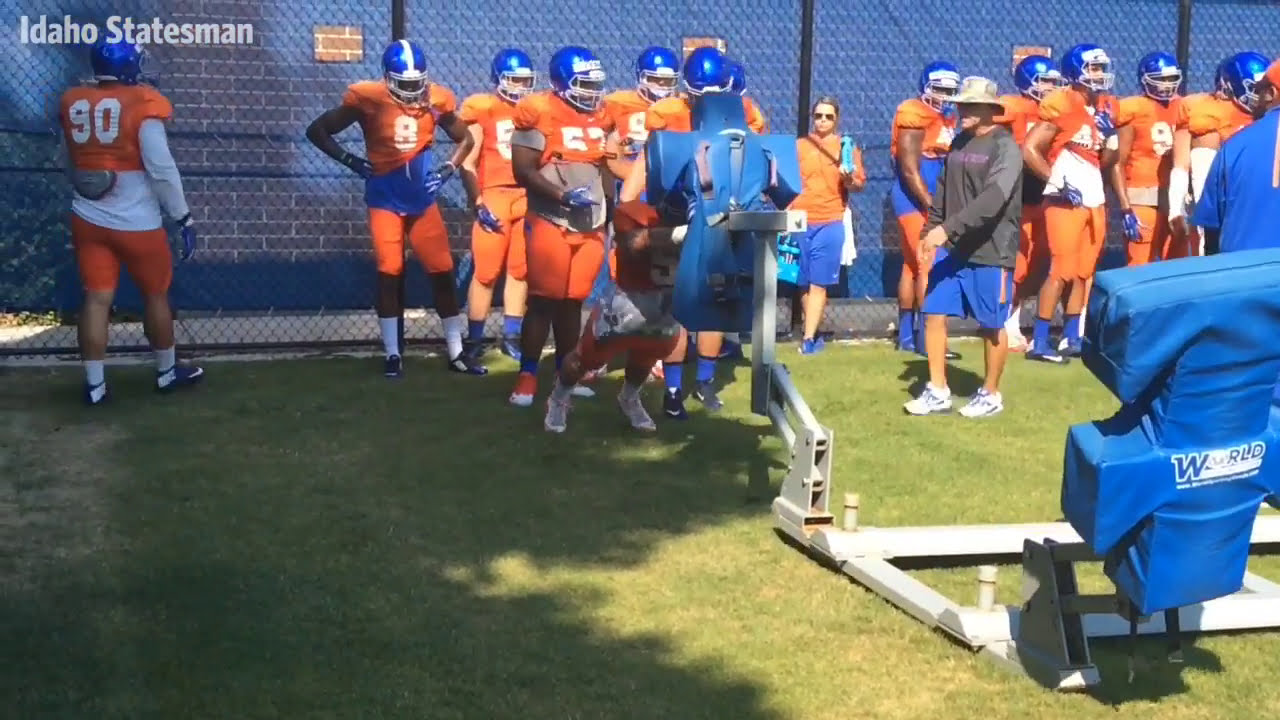The image features the University of Idaho Statesmen football team during a practice session on a green turf field. The team, consisting of about 15 to 20 players, is clustered towards the back of the photo, engaging with blue-cushioned exercise equipment designed for pushing drills. The field itself is partially shaded, with a tree casting its shadow on the left side.

The players are dressed in distinctive orange uniforms that include orange pants and shirts with white numbers and white lettering on both the front and back. They wear blue helmets with writing across the front. Among the visible numbers are 98, 557, 9, and 4. 

Several coaches are present, easily distinguishable by their different attire. One male coach stands prominently in a brimmed sun hat, blue shorts, and a long-sleeved gray shirt, positioned in front of the team. A female coach, wearing an orange jacket and blue shorts, is also seen in the background.

The background features a fenced area with a brick wall or building behind it. The sun is shining from the left, creating shadows from the trees on the field. The exercise equipment, identified by its blue cushions and silver frame, has text on it, including the phrase "Idaho Statesmen" and the word "World."